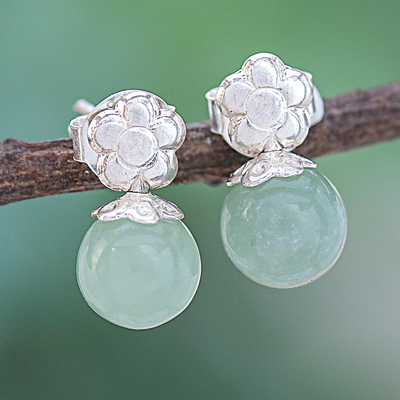This close-up color photograph captures a pair of exquisitely detailed, handmade silver earrings, each featuring an engraved five-petaled flower design. Dangling from the silver flowers are translucent, pale green gemstones that resemble light jade or possibly light emeralds, adding a delicate hint of color. The earrings are artfully positioned on a small, brown twig, imbuing the image with a natural and rustic aesthetic. The background is a tapestry of blurred, various shades of green, which enhances the focus on the earrings, making them the undeniable centerpiece of the composition. The meticulous arrangement and the nature-inspired setting blur the lines between jewelry and art, creating a visually captivating and serene image.